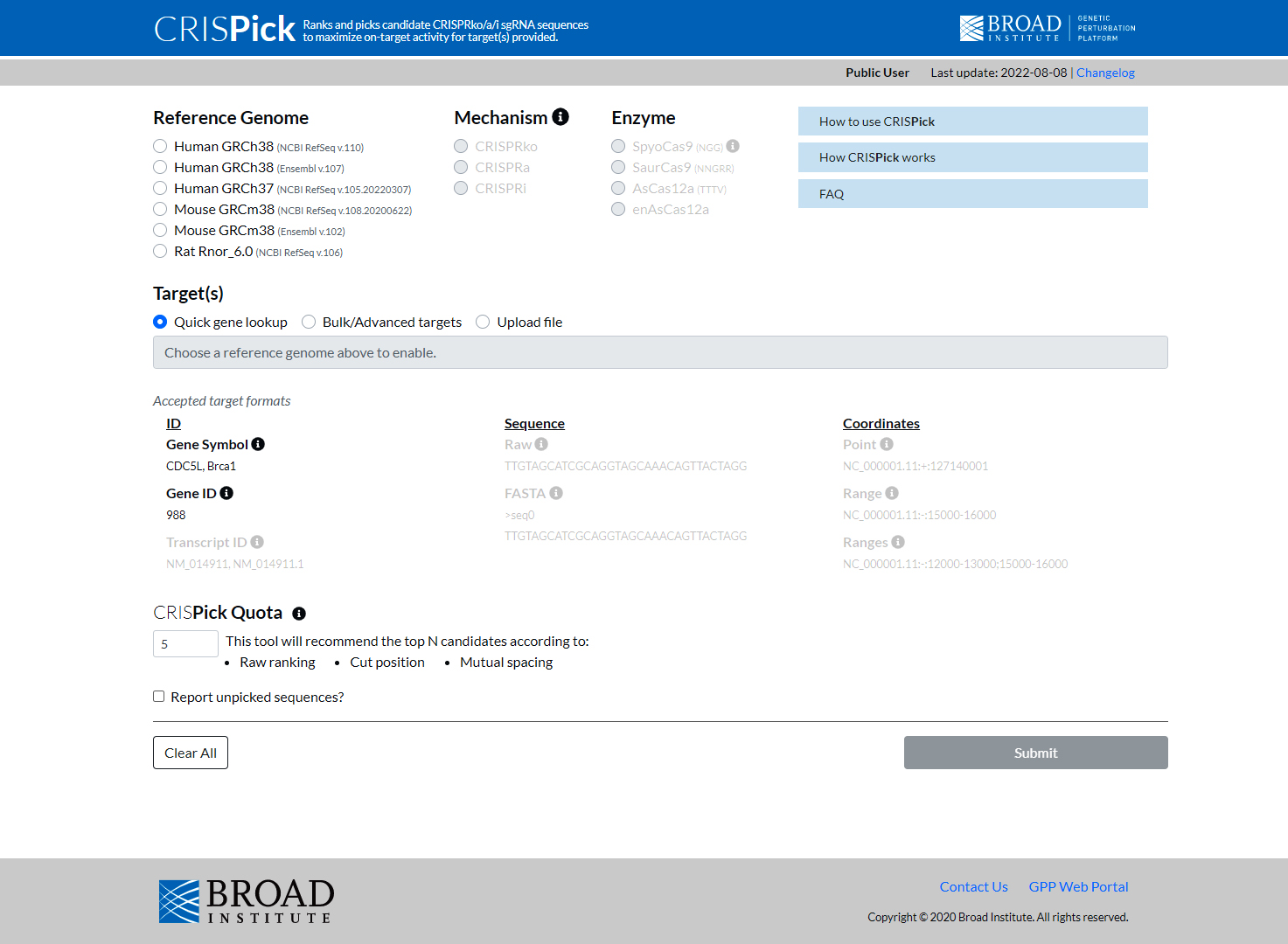A detailed image description of a webpage with various text elements and visual components:

The webpage features a dark blue bezel at the top, containing the text "KRS" in white, followed by the bold white word "PICK." Below this, there are several text sections in white that include "RANKS and PICKS," "CANDIDATE," "CRISPRK," "O," "A/I," and "SG RNA SEQUENCES." This text details the purpose of maximizing on-target activity for targets, indicated by an "S" in parentheses.

On the right-hand side of the top bezel, there is a logo consisting of a white rectangle with blue bands inside it. The logo includes the text "BROAD" in bold white, followed by “INSTITUTE.” Outside the rectangle, there is a white line surrounding the text "GENETIC PERTURBATION PLATFORM" spelled out as "P-E-R-T-U-R-B-A-T-I-O-N."

Following the blue bezel, there is a dark gray bezel on the right-hand side that displays "PUBLIC USER" in bold, and underneath it in dark gray or black text, "LAST UPDATE 2022-08-08," followed by "CHANGE LOG" in hyperlinked blue text.

The main body of the webpage shows various sections and details:

- **REFERENCE GENOME:** Positioned on the right-hand side, this section lists multiple circles (radio buttons) that are currently unselected, each starting with the text:
  - HUMAN (GRCh38, GRCh37)
  - MOUSE (GRCm38, same GRCm38 for another entry)
  - RAT (rnor6.0)

- **TARGETS (S):** This section includes a selected blue circle labeled "QUICK GENE LOOKUP," and subsequent unselected circles:
  - BULK / ADVANCED TARGETS
  - UPLOAD FILE

- **TARGET FORMAT:** Shows a dark gray rectangle at the top with gray text "CHOOSE A REFERENCE GENOME ABOVE TO ENABLE." Below, in white, it details:
  - ACCEPTED TARGET FORMAT
  - ID (in bold black)
  - GENE SYMBOL (underlined, accompanied by a black circle with an "I" inside)
  - Example targets listed as "CDC5L, .BRACA1"
  - Additional identifications including "GENE ID 988," "GENE ID TRANSCRIPT ID (grayed out) NM_014911, NM_014911.1"

Below the target format, there are sequences and coordinates listed:

- **SEQUENCE** (bold black, underlined), showing:
  - RAW
  - TTGTAGCATCGCAGGTAGCAAACAGTACTAGG
  - SPESTA (with an arrow pointing to SEQ0)
  - Another sequence: TTGTAGCATCGCAGGTAGCAACAGTTACTAGG

- **COORDINATES** (bold black, underlined), including:
  - POINT NC_000001.11 +1271140001
  - RANGE NC_00001.11...1500-160000
  - Additional range details

On the left-hand side, there is text in bold that says "CHRISPICK QUOTA." A white rectangle with the number "5" is displayed next to explanatory text about recommending top candidates based on raw ranking, cut position, and mutual spacing:

- REPORT UNPICKED SEQUENCES? (in a separate white square with black text)
- Below, a gray line divides the sections, followed by buttons:
  - A white rectangle with black text "CLEAR ALL"
  - A dark gray rectangle with white text "SUBMIT"

The Broad Institute logo appears again at the bottom, but this time it’s dark blue with white lines, and the text is black. Next to it, two hyperlinked texts "CONTACT US" and "GPP WEB PORTAL" appear, followed by a copyright notice:

- COPYRIGHT © 2020 Broad Institute, all rights reserved, in a dark gray rectangle.

The layout and various sections present are designed to help users navigate and utilize the genetic perturbation platform efficiently.